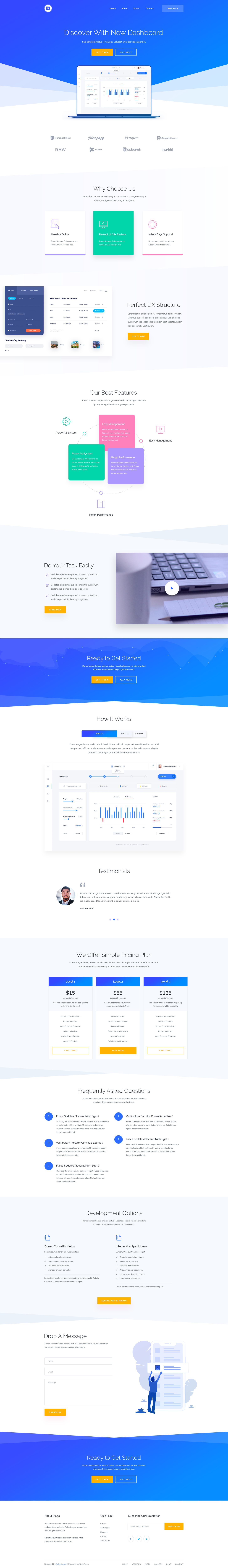The image appears to be an extended composite screenshot of a website, formed by stitching several individual screenshots together. Due to the connection process, it is challenging to decipher specific details. The entire image features various segmented sections laid out in a structured manner.

At the top, there's a banner with a medium bluish color, designed with wavy borders. It contains some white text that is difficult to read. Below this, there's a distinctive yellowish button and an image, likely of a laptop, elongated to fit the design.

Following the initial section, the layout presents four distinct groups of text. Below this segment, three boxes are aligned horizontally: a white box on the left, a green box in the center, and another white box with pink accents on the right. Moving down, two more potential screenshot sections appear, the first being a dark blue box, and the second possibly a table with a white background featuring black numbers and informational text. Additionally, there is another yellow button.

Further down, a triangular arrangement of three boxes is visible, in pink, green, and purple hues, each containing text. Below this triad, there is more text which is suggestive of a video, potentially depicting a laptop keyboard. This is followed by a separator line.

Another segment features a graph-like illustration. Adjacent to this is a profile picture with accompanying text, forming a part of a descriptive narrative. The subsequent section includes three adjacent groups, each characterized by a blue bar above a white text box.

Near the bottom, there's a layout comprising five text groups, arranged as three columns on the left and two on the right. Further down, there is a section with a light blue background and additional text, accompanied by another yellow button and supplementary text. The final element in the image resembles some form of blue vector art.

The overall image is intricately detailed but compromised in readability due to the extensive stitching of multiple screenshots.